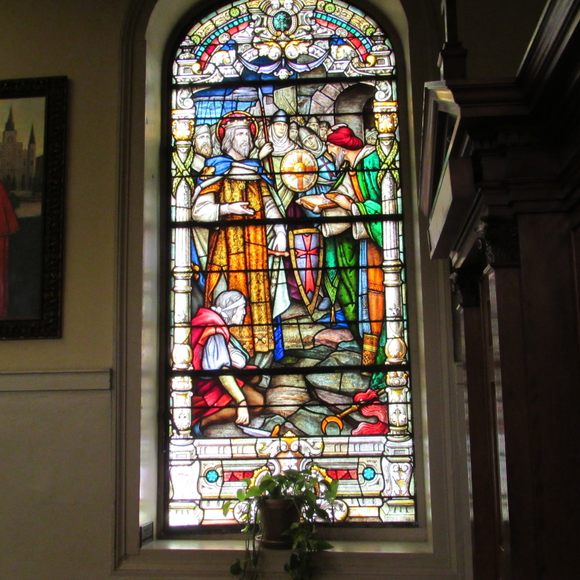The photograph captures a vibrant stained glass window, prominently featuring a detailed depiction of Jesus surrounded by several individuals. The figures are adorned in a variety of vividly colored robes—orange, green, red, and blue—with some dressed in soldier uniforms, distinguished by their helmets and shields. A circular shield and a triangular shield adorned with a cross are particularly noticeable. One man is seen kneeling beside a figure in orange robes, adding depth to the scene.

This stained glass window is framed by an arch-shaped wooden structure, painted white, contrasting with the white-walled surroundings punctuated by veins-like patterns. Intricate cornice-type architectural embellishments add to the elegance of the setting, suggesting a museum-like display rather than a traditional church setting. To the left, a partially visible framed wall art, possibly depicting a castle or towers with a black frame, adds to the decorative ambiance.

A potted plant with lush green leaves sits at the base of the window, adding a touch of nature to the otherwise historical and religious scene. The window and its surrounding decor exude a sense of rich history and intricate artistry.